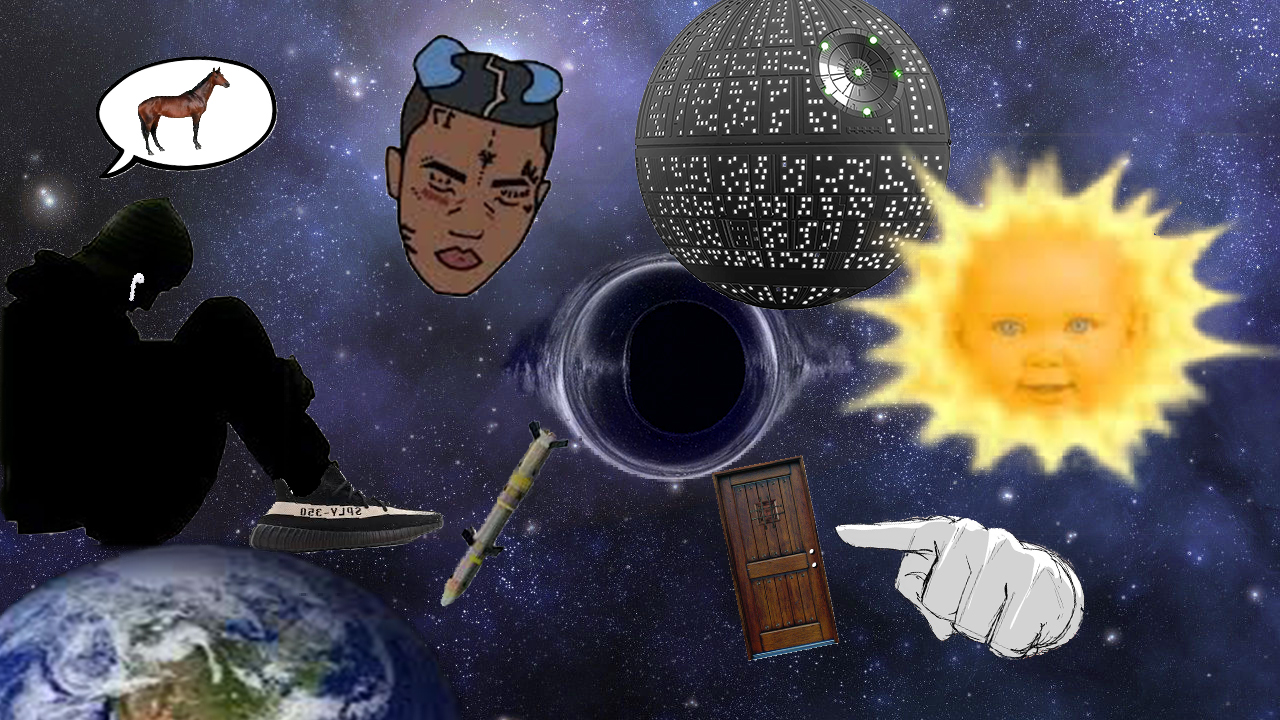The digitally generated collage features a surreal outer space background dominated by a dark blue sky filled with white stars. Central to the image is a black hole with warping effects encircling it. Above it, the iconic Death Star from Star Wars floats ominously. Adjacent to the Death Star, on the left, is a cartoon depiction of a black man's face. To the right of the black hole, the sun contains the face of a baby, reminiscent of the Teletubbies' sun.

Positioned below the black hole is a brown wooden door, with a white illustrated hand pointing towards it, suggesting some enigmatic significance. In the bottom left corner of the image, half of planet Earth is visible, capped by a seated silhouette of an individual adorned with AirPods and tennis shoes, contemplatively hugging their knees. Above the figure is a speech bubble showing a horse, giving insight into their thoughts.

Among the scattered objects is a missile launching from the black hole and various vibrant colors including white, blue, green, brown, orange, yellow, gray, and black, adding to the image's eclectic and chaotic art project feel. No textual elements are present in the composition.